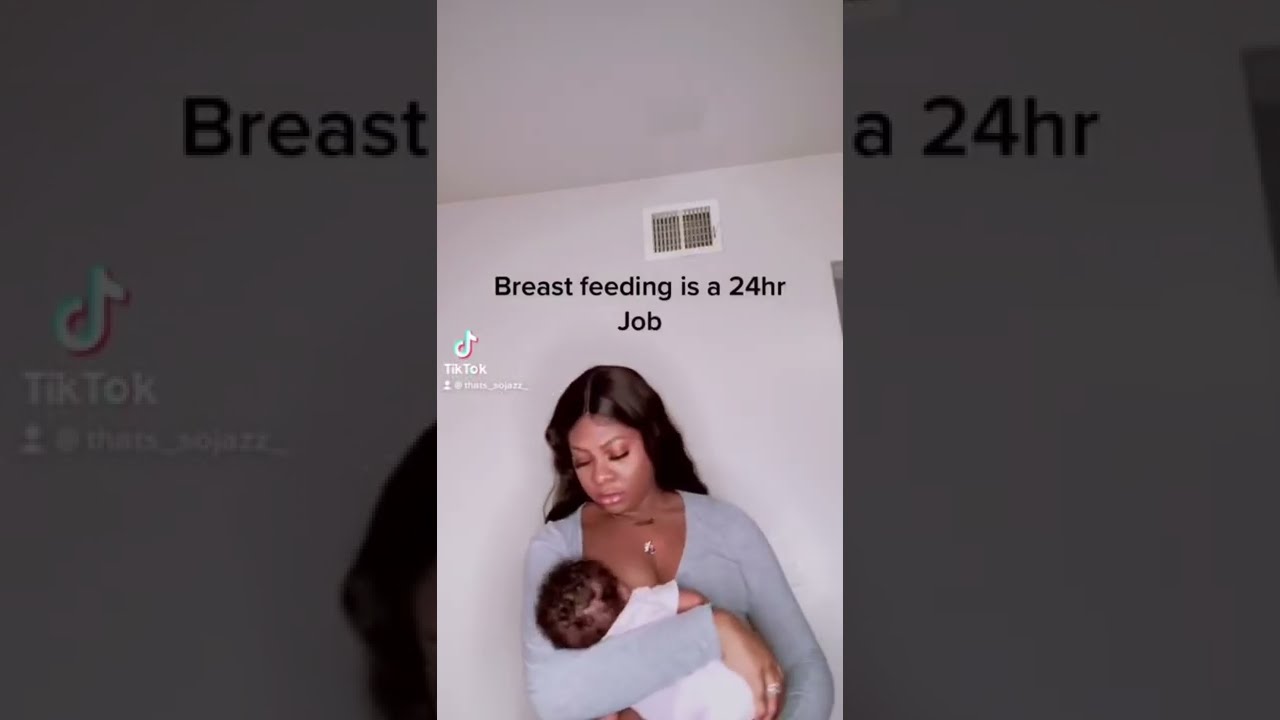This detailed descriptive caption for the image is based on the information provided by the different voice captions:

This is a screen grab of a TikTok video, with the main screenshot centrally focused in a narrow height, suggesting it was recorded on a smartphone. The sides of the video are mostly black with faded visuals, prominently displaying large TikTok logos on both sides. In the center of the image, a young African-American woman with dark brown hair is breastfeeding her baby in a domestic setting, possibly a bedroom with plain gray walls. Above her head, there is a line of black text that reads, "breastfeeding is a 24 hour job." Beside the woman’s head, another TikTok logo is visible with a blurry username of the uploader beneath it. The video’s setting is indoors, and additional details include a white ceiling, a heating or air conditioning vent at the top, and a glimpse of a doorway to the right. The colors present in the image include shades of off-white, white, black, gray, light blue, purple, and brown. The woman and her baby are centered towards the bottom of the image, with the text centrally located, emphasizing the intimate moment captured in this TikTok screenshot.